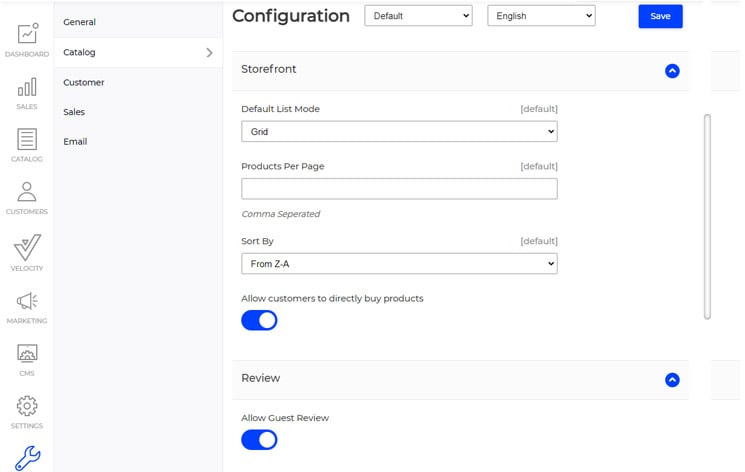In this image, we are looking at a screenshot set against a predominantly white background. At the top center, in bold black text, the word "Configuration" is displayed. To the right of this, there are two dropdown boxes labeled "Default" and "English."

In the top right corner, there is a blue button with the text "Save" in white. Directly below "Configuration," the word "Storefront" appears in gray text. Beneath "Default List Mode," a dropdown box reads "Grid." 

Further down, there is another dropdown box labeled "Products Per Page," followed by a note that says "Comma-separated." 

Below this is yet another dropdown box for "Sort By," showing options from "Z to A." 

Adjacent to this section, gray text reads "Allow customers to directly buy products" with a blue toggle switch indicating that this feature is turned on.

Underneath this section, there is a light gray horizontal line labeled "Review." Below this, in very small gray text, the option "Allow guest review" is displayed with a toggle switch, which is also turned on.